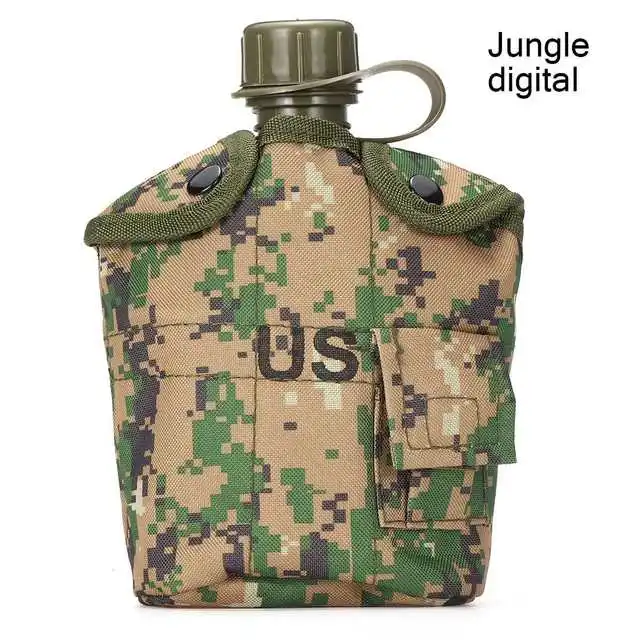The image showcases a military-style water canteen with a dark green cap, encased in a camouflaged cover featuring a Jungle Digital pattern in brown, green, and black. The cover includes two buttons at the top for securing it and boasts the text "US" printed prominently in black on the front. To the right of the text, there is a small velcro pouch for additional storage. The background of the image is white, with the words "Jungle Digital" written in black in the top right corner, indicating the specific camouflage pattern of the product. The detailed and secure design suggests its intended use for military personnel or outdoor enthusiasts.